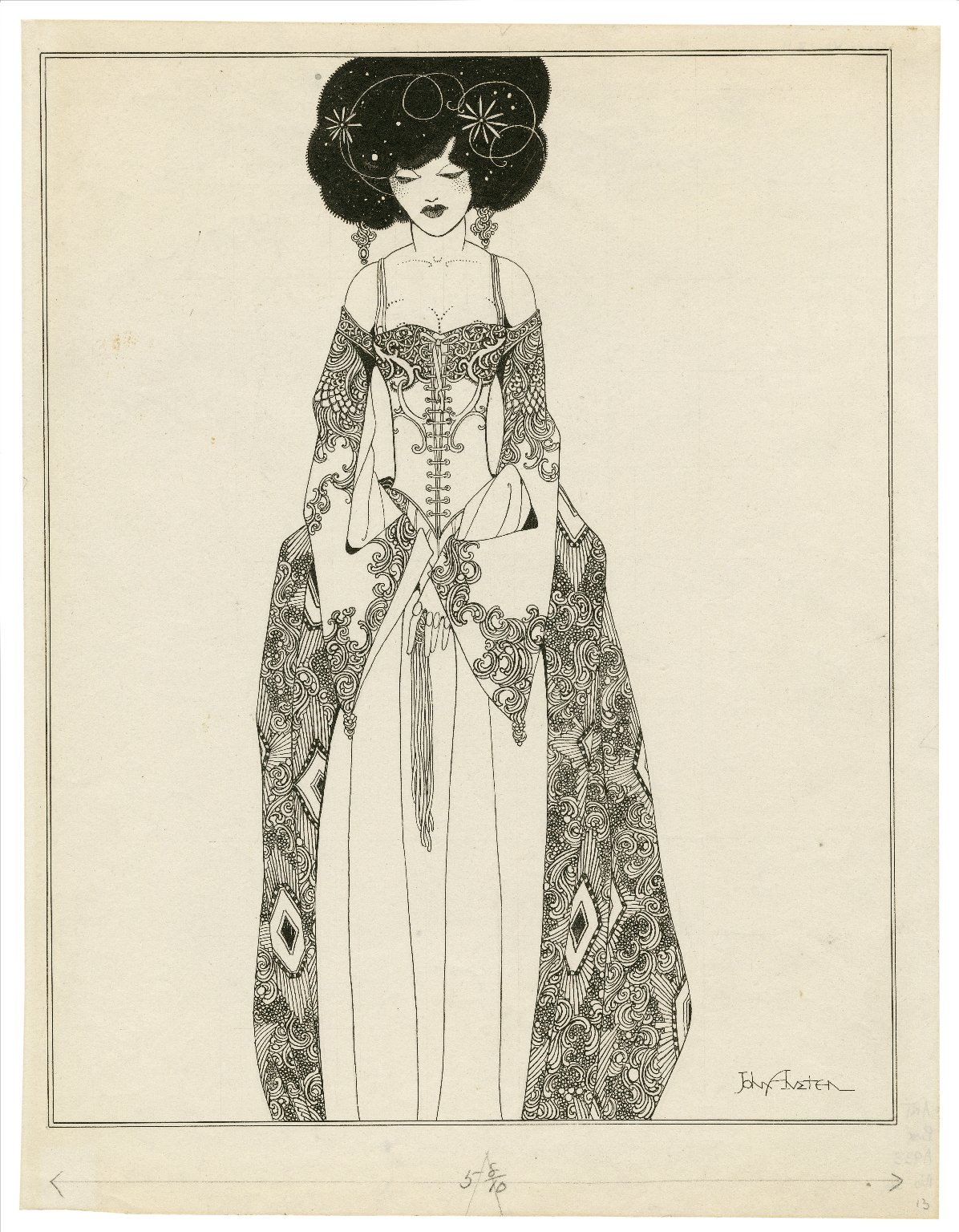This is a highly detailed black and white sketch of a woman, evocative of a vintage postcard. The woman, who has a white complexion, is depicted with voluminous, bold hair adorned with stars and flowers. Her hairstyle is a striking feature, standing up and spreading outwards dramatically. She wears large, dangling earrings that complement her elaborate look. Her attire is an extremely ornate floor-length gown reminiscent of the Victorian era, complete with a corset and spaghetti straps revealing her shoulders and chest. The corset is tied at the middle, accentuating her exaggerated bosom and revealing an ample amount of cleavage. The dress itself is intricately designed with fine-grained swirls, diamond patterns, and an array of other delicate decorations that cover the large bell sleeves and the expansive skirt. The artistry is further highlighted by subtle beads and swirls integrated into the fabric. At the bottom of the sketch, the artist’s signature, "John Beaton," is prominently displayed.